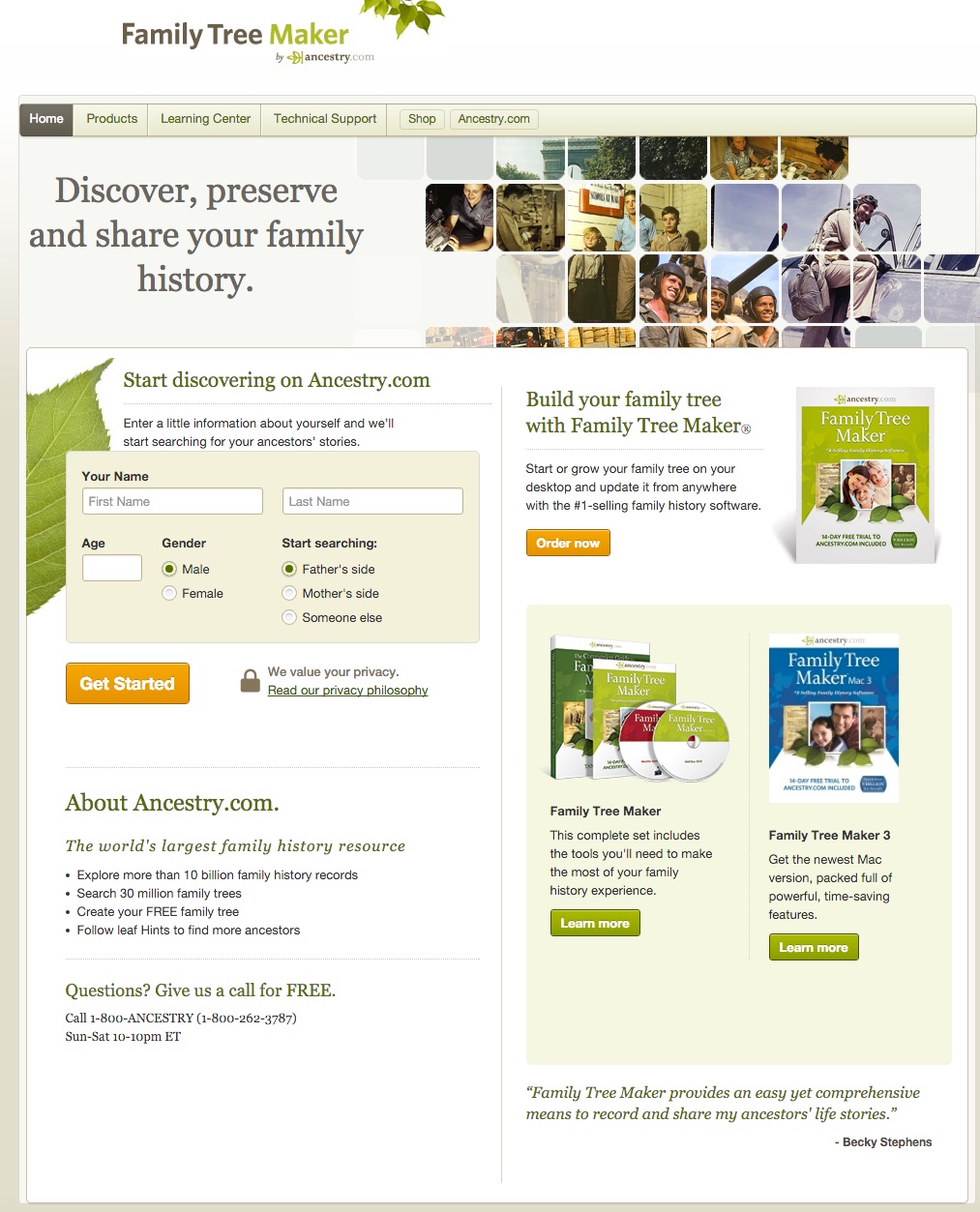This image is a detailed screenshot from Family Tree Maker by Ancestry.com. 

In the upper left corner, the title "Family Tree Maker" by Ancestry.com is prominently displayed. Below the title, a navigation bar features the options: Home, Products, Learning Center, Technical Support, and Shop, with the latter two presented as buttons.

In the upper right quadrant of the image, a collage of smaller images forms a larger mosaic, enhancing the visual appeal. 

On the left side, the text "Discover, Preserve, and Share Your Family History" introduces the main functionality of the platform. Beneath this text, a form titled "Start discovering on Ancestry.com" encourages users to enter their personal information to begin the search for their ancestor stories. This form includes fields for first name, last name, age, and gender, with the example showing the gender selected as male. A large orange button labeled "Get Started" invites users to initiate their family history search, specifically on their father's side.

Further down, additional information about Ancestry.com emphasizes its vast resources:
- The world's largest family history resource.
- Access to more than 10 billion family history records.
- Search capabilities for over 30 million family trees.
- The ability to create a free family tree and follow leaf hints to discover more ancestors.
- A customer service number, 1-800-Ancestry, offering free assistance from Sunday to Saturday, 10 p.m. to 10 p.m.

The right-hand column highlights a disk set and other instructional resources, suggesting there are ample guided materials available to help users navigate and utilize the platform effectively.